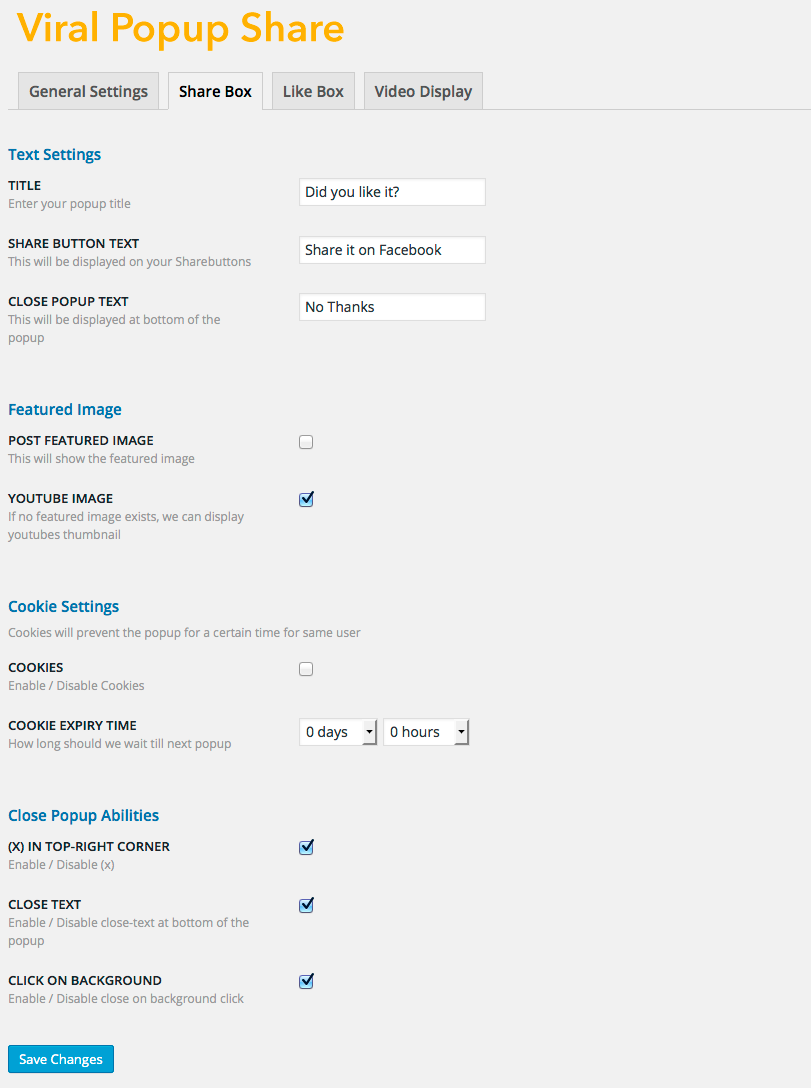The image depicts the settings interface for a "Sharebox" feature, as part of the "Viral Pop-up Share" tool. The rectangular interface, which is taller than it is wide, features a solid gray background. 

In the top-left corner, the title "Viral Pop-up Share" is displayed in a gold-yellow, slightly orange font. Below this title, there are four navigational tabs labeled "General Settings," "Sharebox," "Lifebox," and "Video Display," with the "Sharebox" tab currently selected.

Within the "Sharebox" settings, various configuration options are presented. The section header "Text Settings" is highlighted in a blue font. Underneath this, there are fields for customizing the text of the share button and close pop-up button:
- The "Share Button Text" field contains the entry "Share it on Facebook."
- The "Close Pop-up Text" field displays "No thanks."

In black font, the title for the pop-up reads "Did you like it?" 

Further configurable options are grouped under sections for "Preferences," "Featured Image," "Cookie Settings," and "Close Pop-up Abilities," though specific details for these sections are not filled in.

At the bottom-left corner, a blue box with white font inside provides a "Save Changes" button. 

Overall, the image shows an individual customizing the settings for a pop-up window intended to prompt users to share a post, image, meme, or other pieces of content on Facebook, while also offering the option to decline with a "No thanks" response.